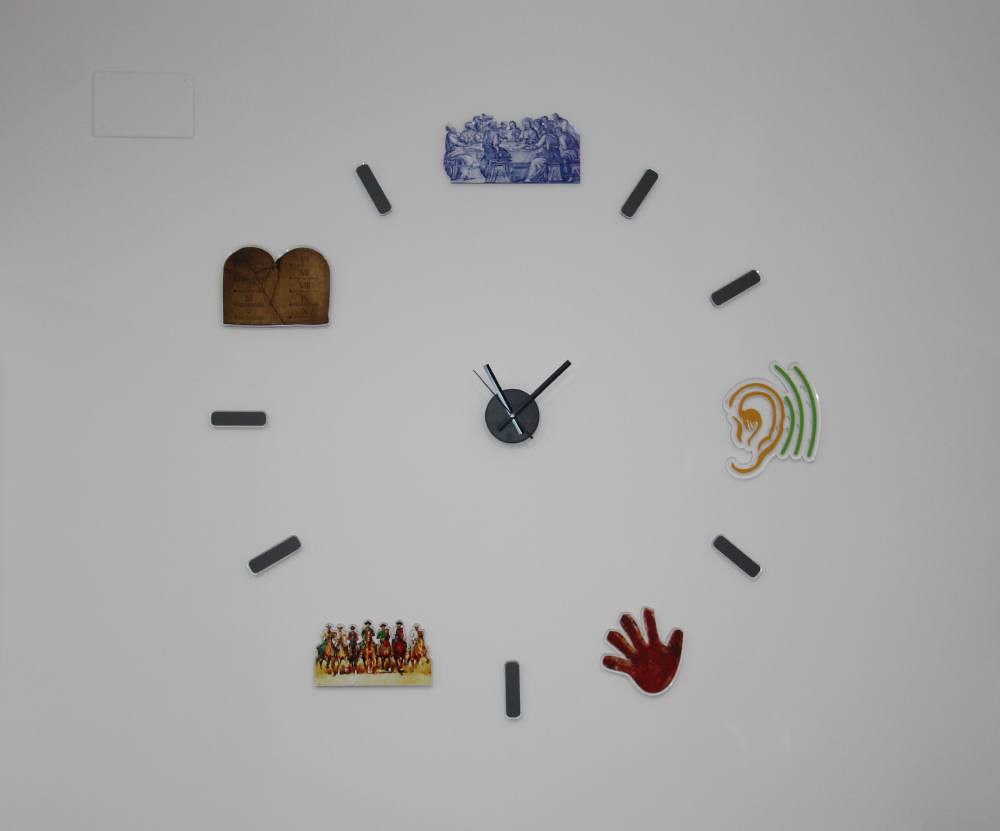This uniquely designed wall clock replaces traditional numbers with a mix of religious and pop culture icons, creating a visually intriguing and eclectic piece. At the 12 o'clock position, a blue image depicts the Last Supper. Both the 1 and 2 o'clock positions are marked by simple lines. The 3 o'clock spot features an ear surrounded by green lines, symbolizing the reception of sound. At 4 o'clock, there is another line. The 5 o'clock position is illustrated by an image of a hand displaying five fingers. A single line marks the 6 o'clock position. At 7 o'clock, an image of the seven cowboys from "The Magnificent Seven" riding their horses is displayed. The 8 and 9 o'clock positions are each marked by lines. The 10 o'clock spot showcases the stone tablets of the Ten Commandments, and at 11 o'clock, there is a single dot. This clock creatively combines elements from religion and popular culture, resulting in an unconventional and visually striking wall piece.